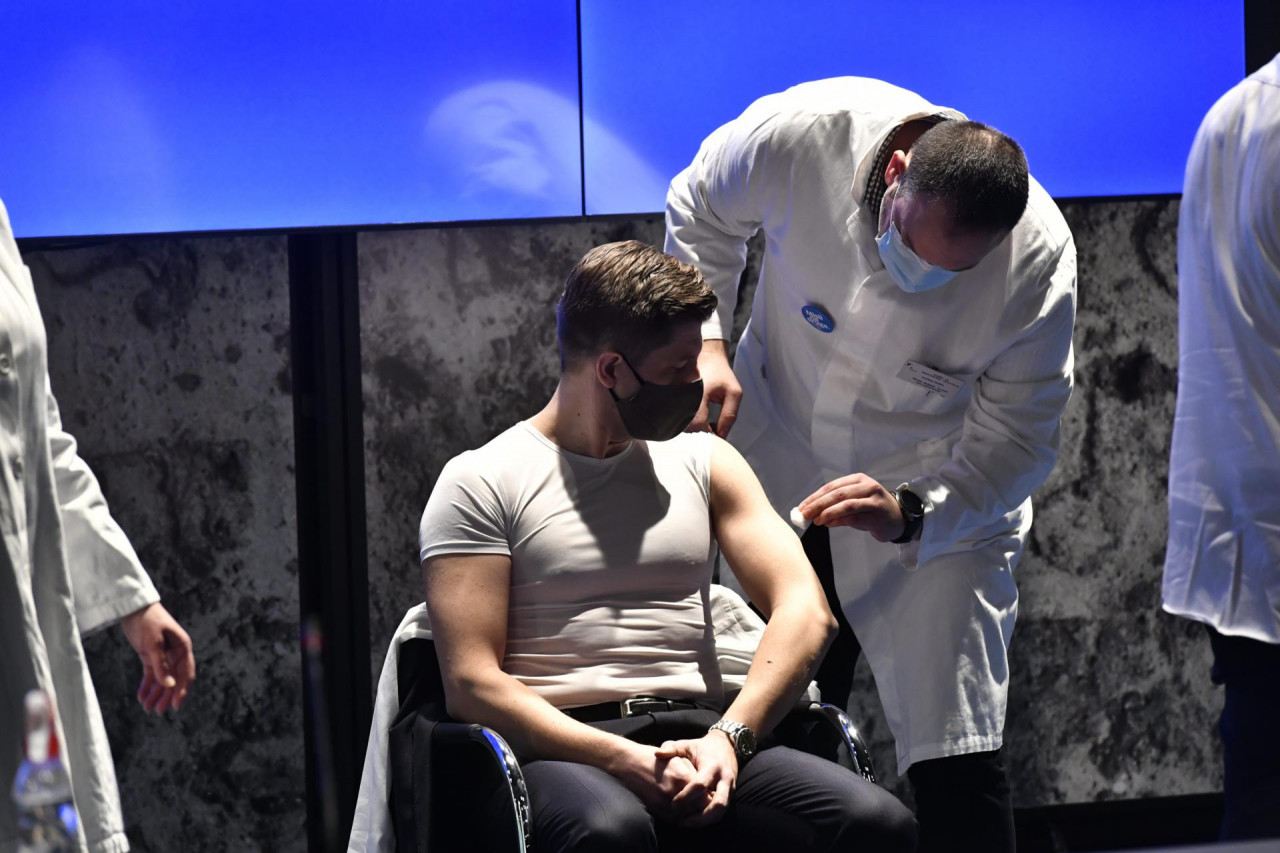In this color photograph, we observe a young man with a muscular build seated in a chair, attentively looking down at his left upper arm. He is dressed in a tight, tan short-sleeve t-shirt, with the left sleeve pulled up to expose his arm. His ensemble is completed with black pants and a black belt. A watch adorns his left wrist, and his hands are neatly crossed in his lap. His face is partially obscured by a black mask, and he has short, dark hair. 

Standing beside him is a man in a white jacket, also wearing a mask, who appears to be preparing to administer a vaccine. The man in the white jacket is gazing down at the young man's arm and is holding a cotton ball, likely swabbing the area in preparation for the injection. To the right of the central figures, we see the back of another person clad in a white jacket, and on the left, only the arm of an additional individual similarly dressed.

The backdrop of the scene is a gray wall with a glass window positioned above, through which the daytime blue sky and soft, swirling white clouds are visible, adding a touch of serenity to the clinical setting.